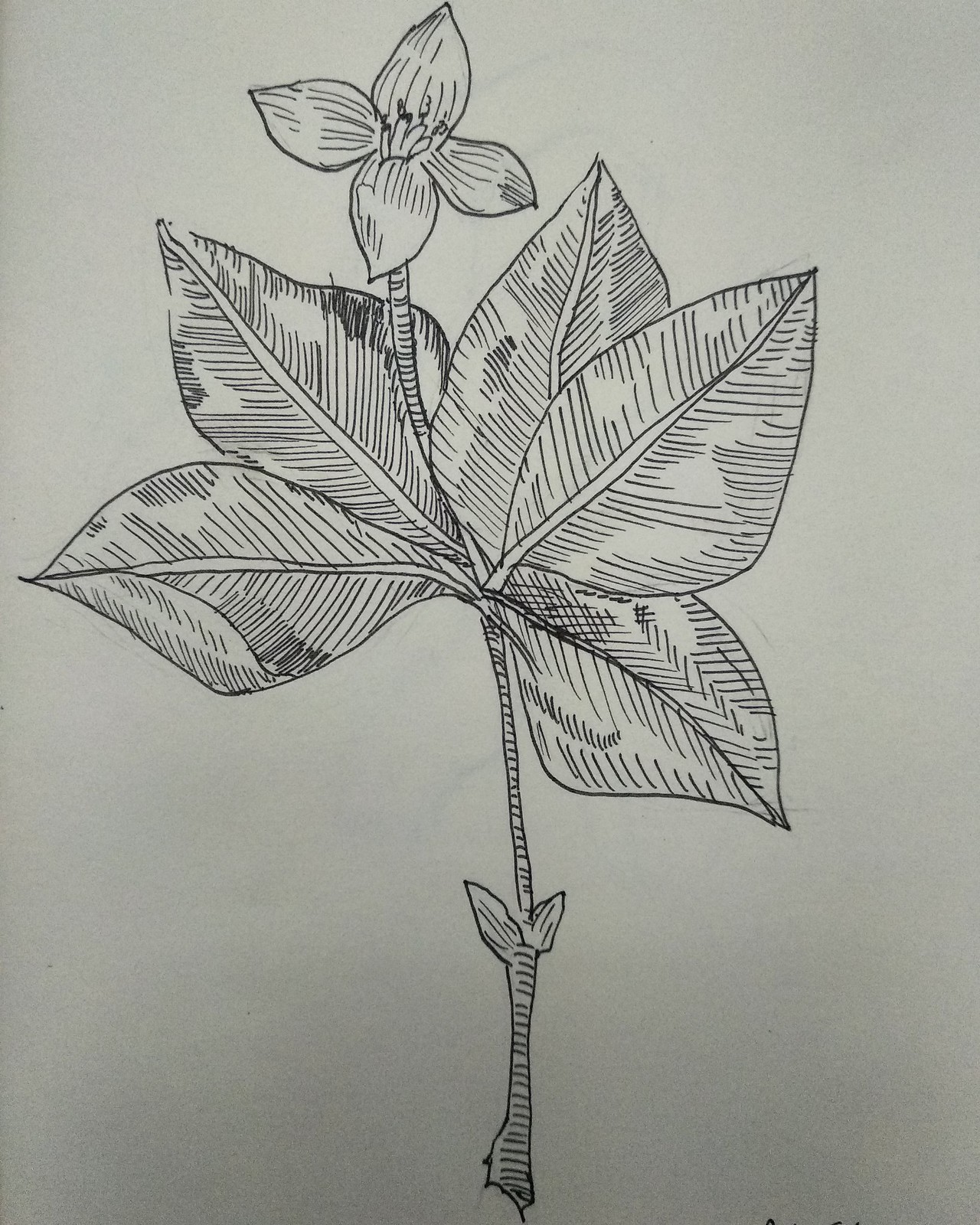This image features a detailed drawing on a sheet of white printer paper, created with a black pen. The drawing depicts a plant with a slender stem that starts at the bottom, where two small leaves are attached. As the stem ascends, it branches out into three larger, intricately-drawn leaves. At the very top, the stem culminates in four delicate flower petals, complete with inner lines that likely represent stamen and pistil, hinting at seed dispersal. The artist skillfully employs line shading techniques, using varying lengths and densities of lines to create depth and texture. Additionally, negative space is expertly utilized to highlight certain areas, giving the drawing a three-dimensional and strikingly realistic appearance.